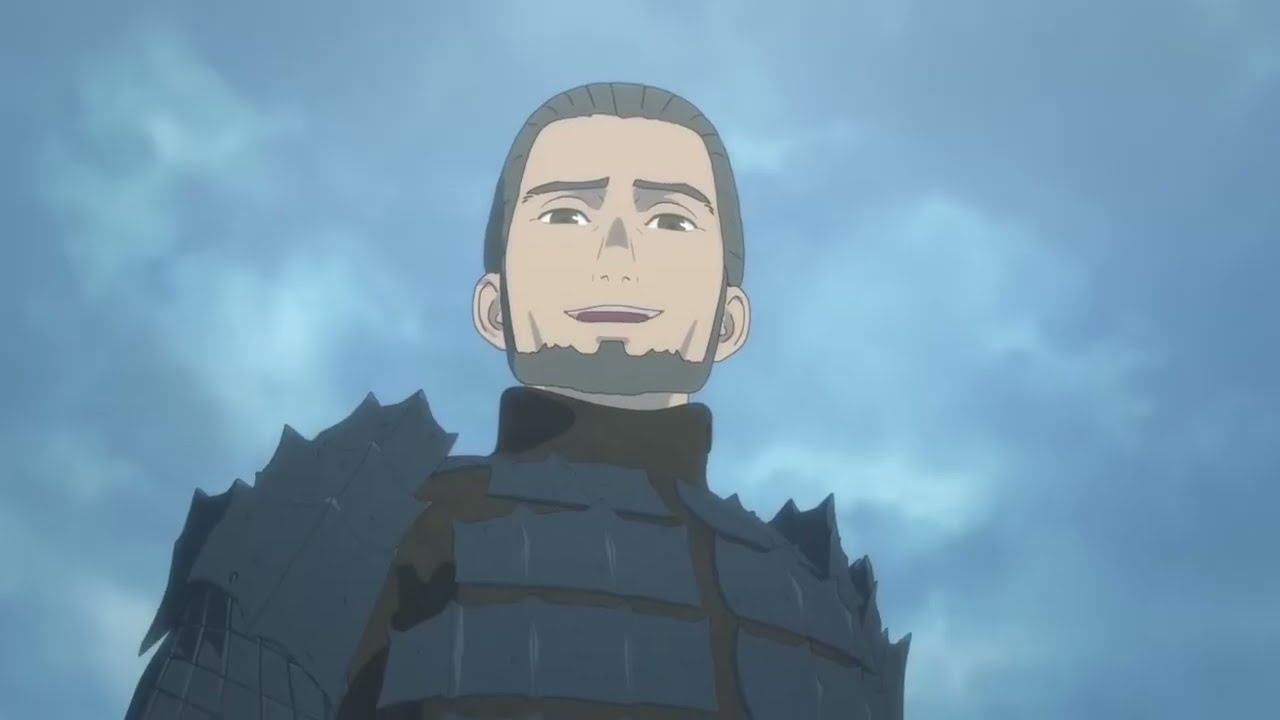In this detailed and descriptive single caption, we'll merge the shared and repeated aspects while emphasizing the strongest and most vivid details from each individual caption.

---

The image captures a still from an anime, featuring an older male character who exudes confidence and strength. He has slicked-back gray hair, complemented by a grey chin beard and thick eyebrows. His piercing gray eyes gaze down at the viewer, creating a perspective as if the viewer is laying on the ground looking up at him. The man wears intricate armor consisting of a black undersuit with a high collar that shields his neck, overlaid with dark blue, scale-like plates that give it a spiky, mountain range appearance across his chest and shoulders. Despite the heavy armor, he smiles warmly and confidently, suggesting a sense of victory or reassurance. The background depicts a dramatic, cloudy sky with varying shades of dark blue and gray, enhancing the intense and triumphant ambiance of the scene. This fearless, battle-ready character appears to be addressing his troops, perhaps after a victorious conquest, epitomizing the essence of a seasoned and successful warrior in the world of anime.